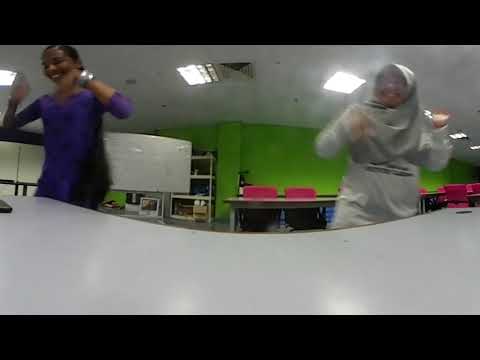This photograph captures a lively moment of two individuals, presumably in a classroom setting, who appear to be dancing and enjoying themselves. On the left, there is a woman with black hair, adorned in a long, elegant purple and black dress with silver jewelry. She has a smile on her face and her arms are raised to shoulder level, bent at the elbows. On the right, another woman is seen wearing a light gray hijab along with a white t-shirt underneath. Her outfit seems to be completed with gray clothing, possibly a sweatshirt and pants. She too is smiling and has her arms positioned similar to the woman on the left. 

The backdrop is a vibrant lime green wall, adding a fresh and energetic vibe to the scene. The white ceiling above is fitted with numerous square-shaped fluorescent lights that illuminate the room brightly. Magenta or pink chairs are placed in front of the lime green wall, along with a table that suggests the setting is possibly a classroom. In the foreground, a white table or counter can be seen, serving as the surface where the photograph was likely taken.